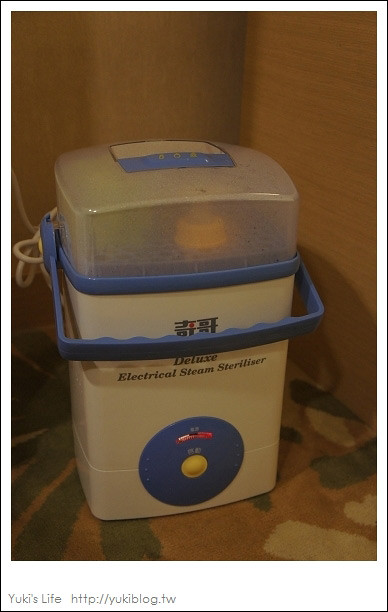The image captures a deluxe electrical steam sterilizer in a corner of a room with two brown walls and a camouflage-patterned floor. The rectangular device features an opaque, dome-shaped lid with a blue rim, and a folded blue handle on top. Inside the foggy lid, vague shapes resembling baby bottle tops and nipples in yellowy-orange are visible. A prominent blue circle with a smaller yellow circle and a thin red stripe is located in the bottom center of the sterilizer. The device bears the label "deluxe electrical steam sterilizer" along with an Asian script above it and a partially visible email address “http://yukiblog.tw” below. To the left of the item, a thin white cord extends outward. The photograph, taken indoors in portrait orientation, is dimly lit, contributing to a muted ambiance.